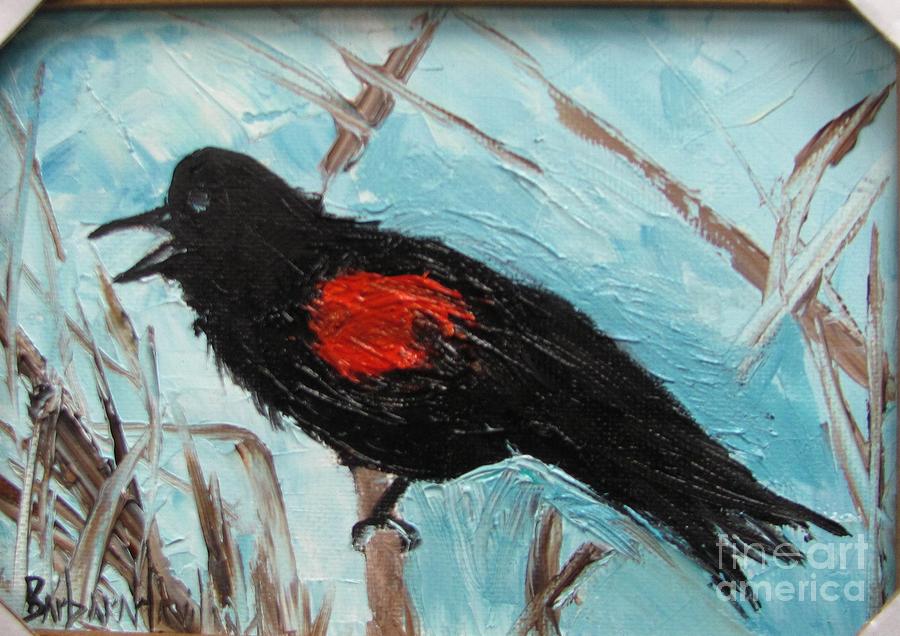This is a detailed oil painting that depicts a black crow with a long beak and striking red spot, suggestive of blood, on the center of its body. The bird is facing towards the left, with its beak slightly open, and clasping a small stick with its visible talon, while fragments of wood and cloth surround it. The thick, three-dimensional brushstrokes create a textured background that is predominantly a mix of turquoise blue, with hints of other colors resembling twigs or greenery. The painting features the artist's signature, possibly reading "Barbanto" or "Barbian," in black at the bottom left corner. Overlaying the bottom right corner is the semi-transparent text "Fine Art America."